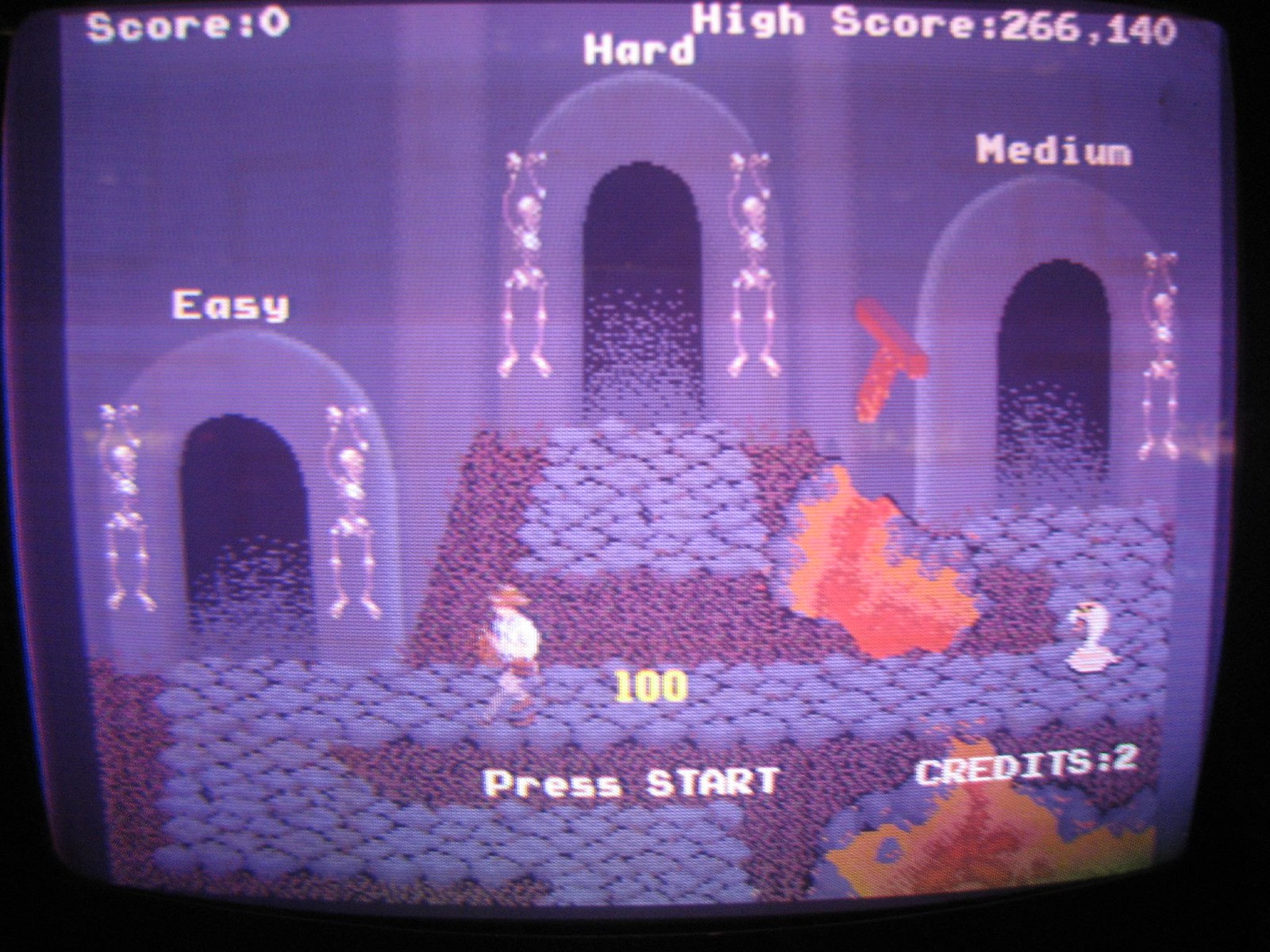The image is a screenshot from a video game, prominently featuring a predominantly purple background reminiscent of the game's level design. Dominating the scene are three large, arch-shaped portals, each in varying heights and uniformly hued in purple. These doors are adorned with white skeleton decorations on both sides, adding a touch of eerie ambiance.

The leftmost door, marked as "Easy" in white text above it, is the shortest. The central, tallest door is labeled "Hard" in white, suggesting a more challenging level. The right door, of medium height, is inscribed with "Medium" in white text, indicating an intermediate difficulty.

In front of these doors stands an avatar resembling Indiana Jones. The character is outfitted in a white shirt and a distinctive brown hat, enhancing the adventurous aesthetic. Below the avatar, "Press Start" is prominently displayed in white, with the number "100" in yellow above it, possibly signifying a score or level indicator.

Additionally, the ground showcases a detailed path, guiding players towards selecting a door to enter, hinting at the interactive nature of the game. The overall scene is rich with intriguing details and beckons the player to embark on a thrilling adventure.